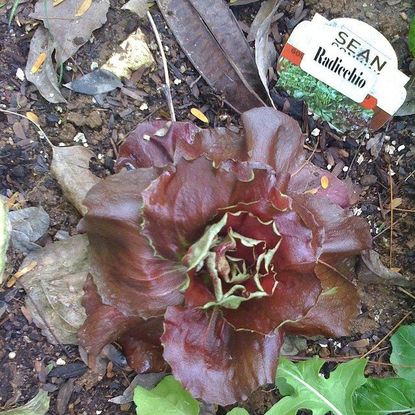This is a square-shaped photograph taken from a top-down view, capturing a radicchio plant that remarkably resembles a flower in its form and color. The plant features several layers of deep purplish-red leaves with green edges around the smaller, inner leaves. These leaves are densely packed in the center and fan out towards the edges. The ground surrounding the radicchio consists of dark brown soil mixed with mulch, scattered with dead leaves and other debris. In the bottom right corner, fresh green leaves from a nearby plant are visible, adding a touch of vibrancy to the image. Additionally, in the upper right corner, there is a small white paper label with the text “SEEN READY GEO,” misreading what actually says "radicchio," indicating the plant type.